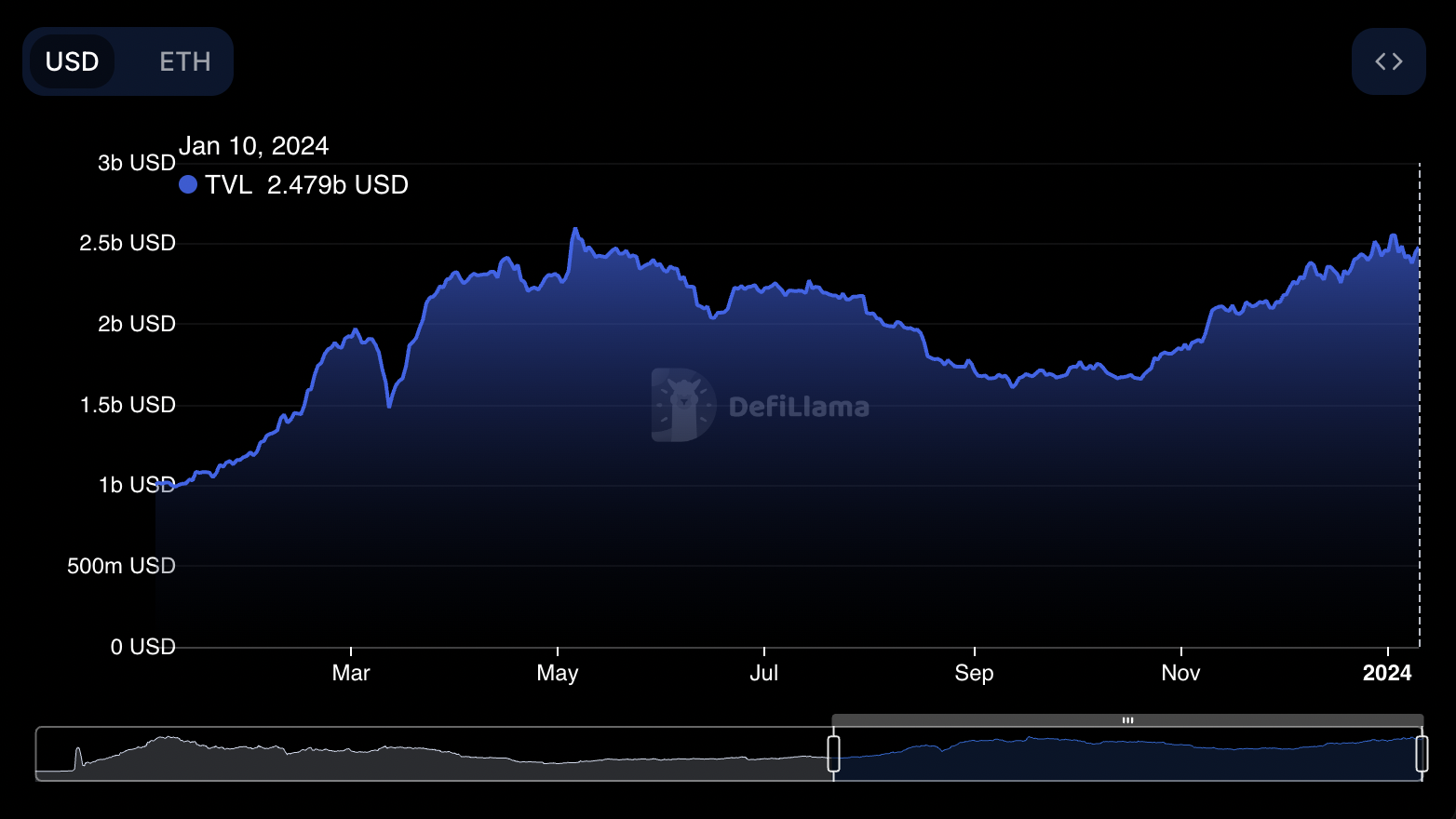The image features a graph set against a black background, showcasing an ombre effect where the graph transitions from dark blue at the top to black towards the bottom, framed in neon blue. In the top left corner, "USD" is prominently displayed in capital white letters, indicating selection with a navy rectangular icon nearby, displaying "ETH" in light gray. This is a representation of currency choices, with USD being the active selection due to the highlighted black background.

Along the left axis, several white labels indicate monetary values in BUSD (Billion USD) descending from 3BUSD, 2.5BUSD, 2BUSD, 1.5BUSD, 1BUSD, 500MUSD to 0USD at the bottom. The horizontal axis features month abbreviations "MAR," "MAY," "JUL," "SEP," "NOV," ending with a bold "2024" on the far right. The far-right edge of the graph is delineated by a vertical border consisting of gray dashes.

At the top right section of the graph, a grayish area displays icons with arrowheads pointing left and right, suggesting navigation options. Below the graph, there's an interaction component for user adjustment, consisting of a small oval slider with two extending lines. The left segment of this slider area is gray with a white border, while the right segment sports a dark bluish-black hue bordered by ultraviolet blue. Above this slider, a gray strip with three central white lines runs horizontally. Each month listed along the top center includes a minor white demarcation line, enhancing the timeline clarity.

In summary, the graph presents detailed visual and interactive elements that depict financial data over specified months, offering intuitive navigation and user adjustments.